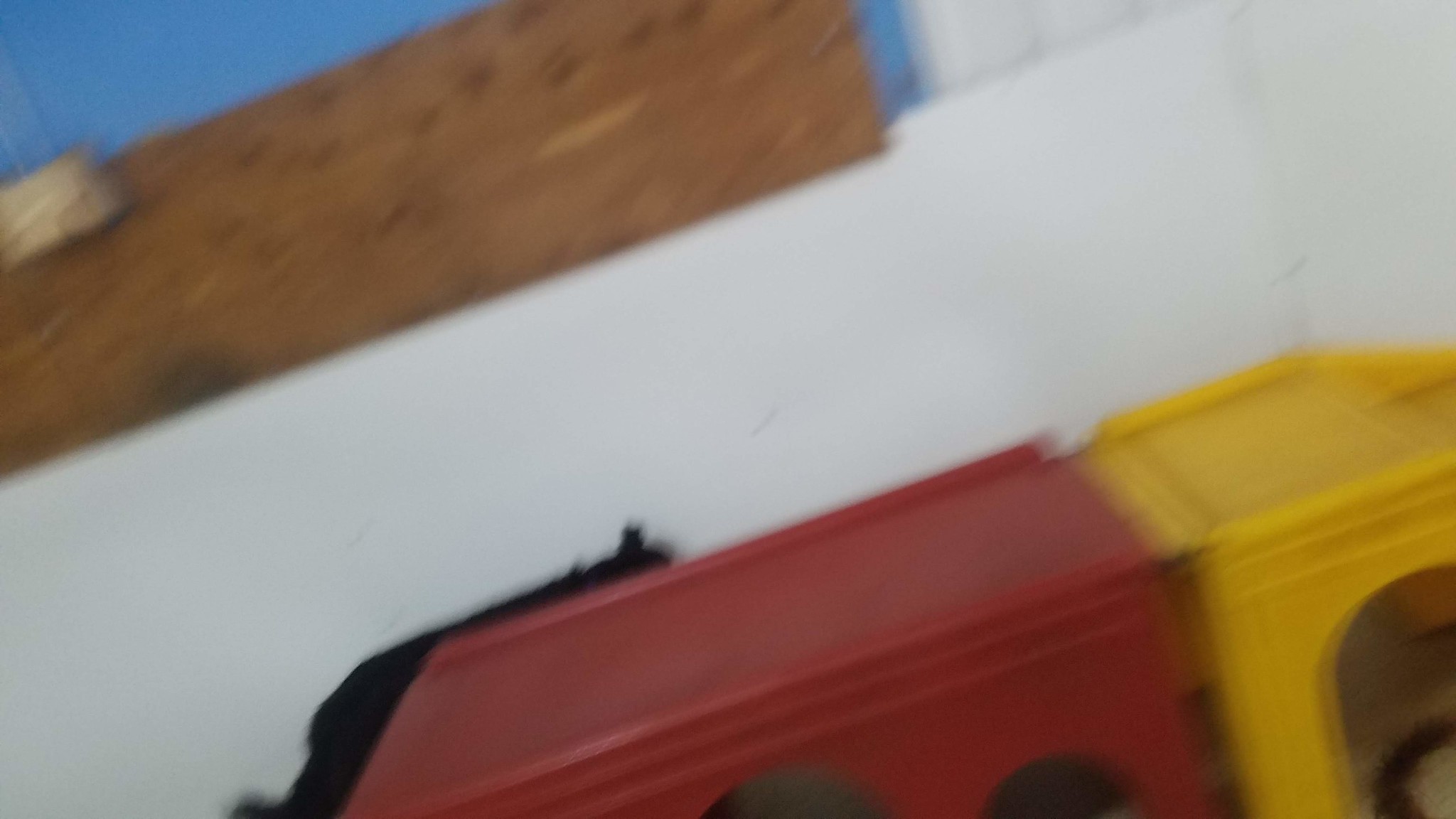This image is very blurry and difficult to decipher, lacking a clear focal point. At the bottom of the image, there is a red and yellow plastic object, possibly a toy or part of a child's playset. The yellow portion is flat on top with ridges around it and has a square shape with cutouts that suggest it could be part of a toy bridge or roadway. The red section also has several cutouts facing the front, adding to the toy-like appearance. Above this object, there's a white wall or shelving unit. Behind it, a wooden board or piece of plywood stretches from the left side to the upper right side, partially obscuring a medium blue wall in the background. The board appears to be about two feet wide and rests on the white wall, suggesting some depth. The overall composition tilts at an approximate 45-degree angle from the lower left to the upper right, adding to the disorienting and blurred nature of the image. There’s also a barely visible black object between the white wall and the red section, possibly another part of the toy or a small, indiscernible item.